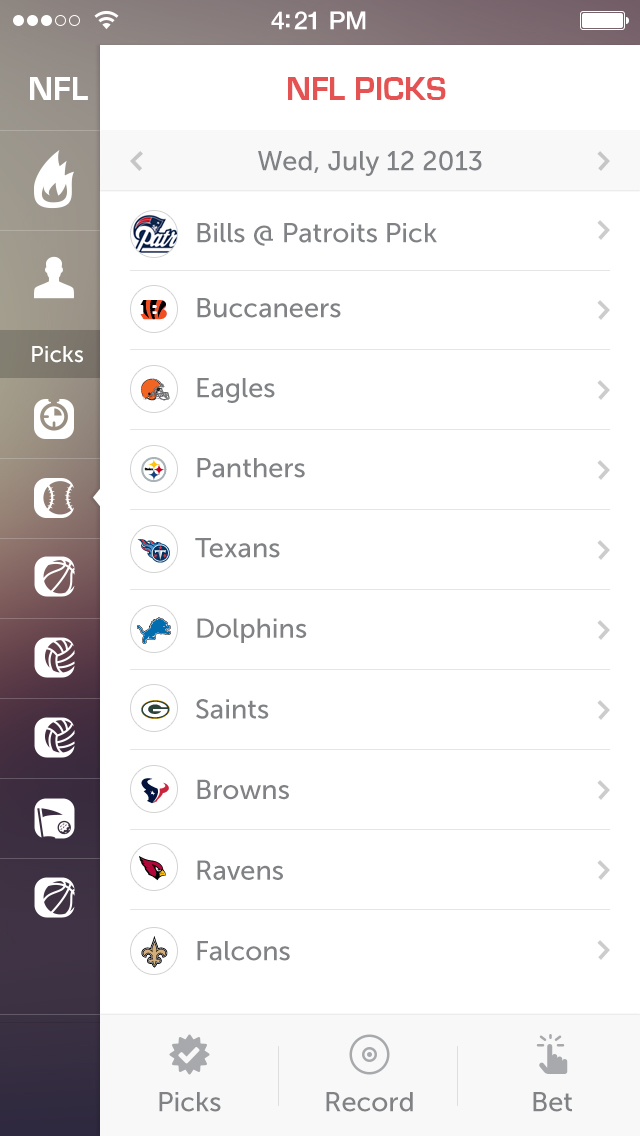This image depicts a screenshot from an unspecified mobile app, possibly either Android or iOS. At the top of the screen, the status bar shows a fully charged battery icon, the current time as 4:21 PM, and a cell signal strength indicator with three out of five bars illuminated. Additionally, a Wi-Fi icon indicates a strong connection.

The left side of the screen features a vertical column of clickable icons. The first icon is labeled "NFL," identifying the mobile application as being related to the NFL. Following this are several icons representing different sports categories or sections, including:
- A head profile icon
- A globe icon
- A baseball icon
- A basketball icon
- Two volleyball icons

Dominating the right side of the screen is a large white area with "NFL Picks" displayed prominently in red text. Below this header, the date for the NFL picks is shown as Wednesday, July 12, 2013. Underneath the date, a list of NFL team match-ups is presented with team names and logos. The first match-up listed is "Bills at Patriots," featuring the Patriots logo. Following that are several other team pairings:
- Buccaneers and Eagles
- Panthers and Texans
- Dolphins and Saints
- Browns and Ravens
- Falcons